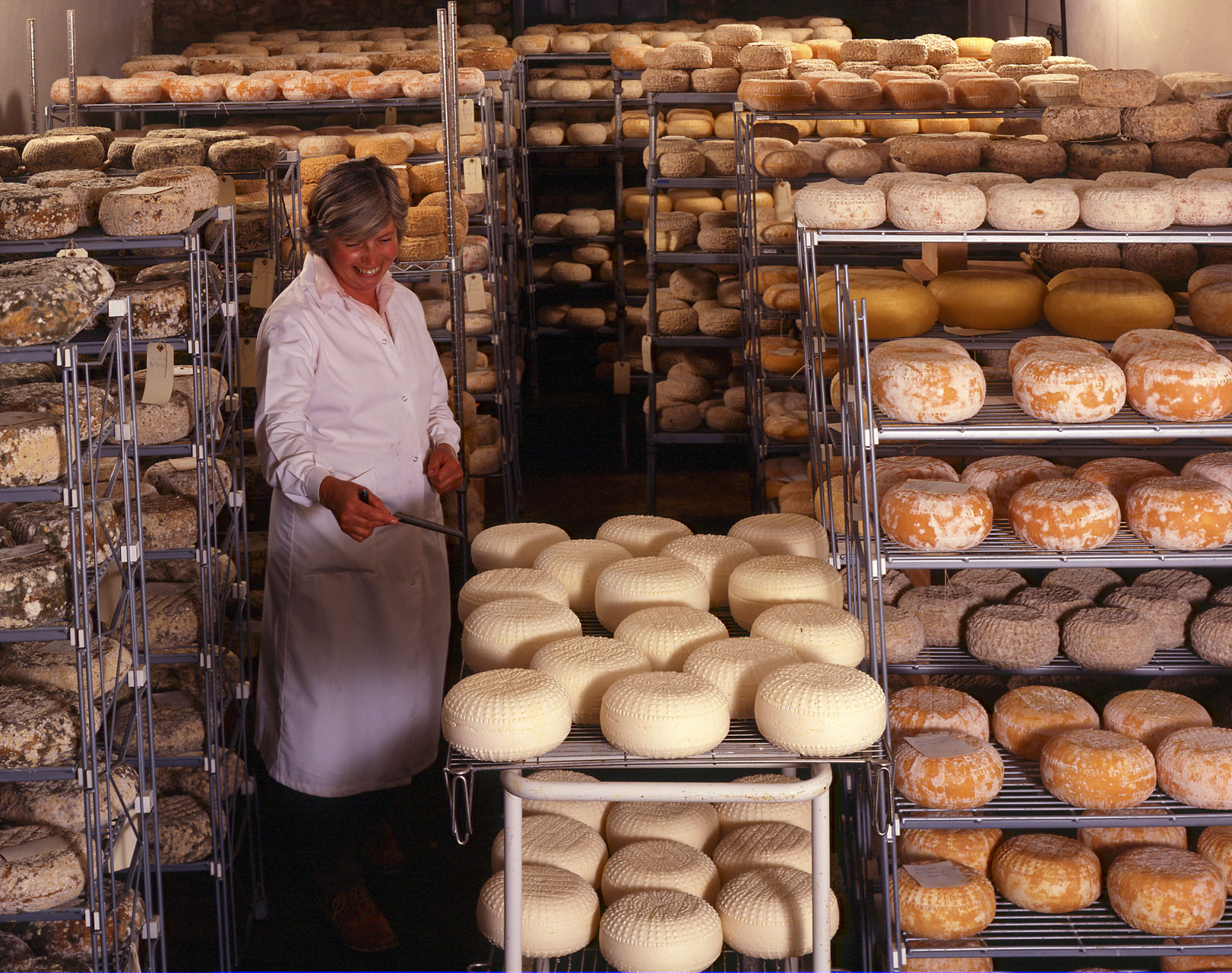The image captures a bustling bakery kitchen filled with rows of gray metal shelving units, each shelf loaded with an assortment of baked goods. The shelves stretch into the background, showing an extensive collection of round bread items, many of which are orange or brown, some dusted with white powder that appears to be powdered sugar. Positioned towards the left side of the photo is an older woman with short grayish-brown hair, wearing a white long-sleeve smock, similar to a lab coat. She stands amidst the shelves, holding a narrow gray object in her right hand, seemingly taking the temperature of several beige circular baked goods on the top rack of a shelving unit. Her presence and careful inspection contribute to the sense of meticulous attention in the busy bakery scene, surrounded by shelves brimming with various breads, cakes, and donut-like treats.